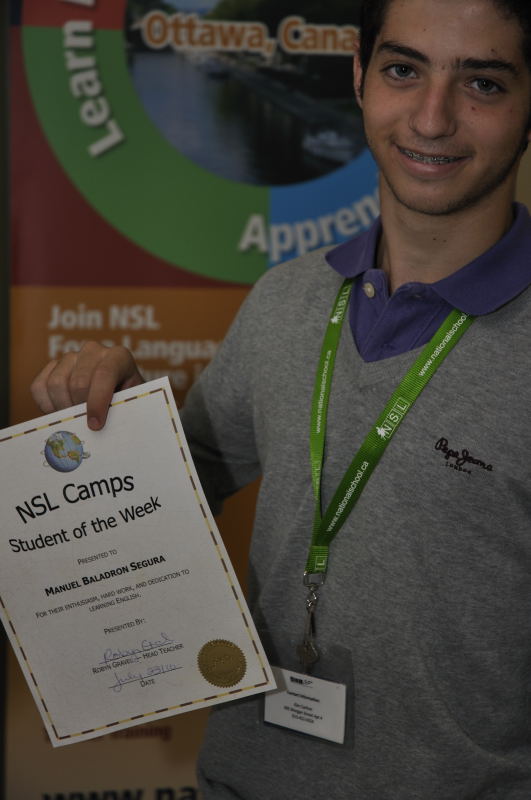This image features a smiling teenage boy named Manuel Boladran-Segura, who is proudly holding up a certificate. He is wearing a gray sweater over a purple collared shirt, and a name tag is hanging around his neck on a green ribbon. The certificate in his right hand reads "NSL Camps Student of the Week," and it has a gold seal in the lower right-hand corner, set against a white background with black text. The backdrop is vibrant and colorful, displaying large text that spells out "Ottawa, C-A-N-A." In the margin, there are words such as "learn" and "A-P-P-R-E-N," along with a sign that says "join NSL" in white letters on an orange background, creating a lively and engaging atmosphere.